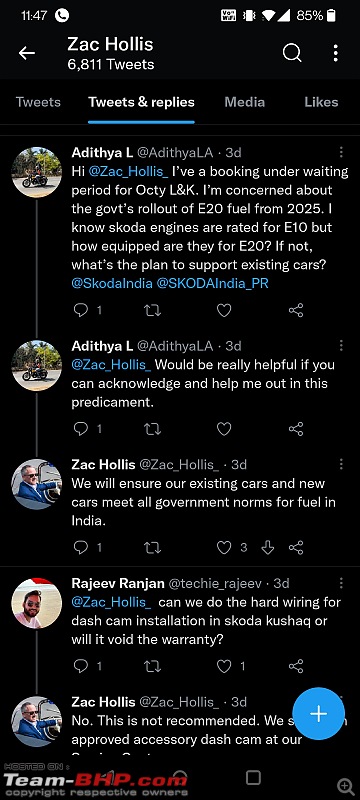The image displays a smartphone screen against a black background, highlighting the "Tweets and replies" section of a user's Twitter profile. At the top left of the screen, the time reads 11:47, along with a filled-in phone icon indicating a voicemail message. The battery level is at 85%, and the device shows full signal bars. The user's name, "Zach Hollis," is prominently displayed in white text, and he has 6,811 tweets. To the left of his name, an arrow points back to the previous screen.

Below his name, various navigation options are visible: Tweets, Tweets & replies, Media, and Likes, with the "Tweets & replies" tab highlighted and underlined in bright blue. The main content features a conversation with a user named Adithya L., whose avatar icon depicts a motorcycle. Adithya's tweet reads:

"Hi Zach Hollis, I've a booking under waiting period for October L&K. I'm concerned about the government's rollout of E20 fuel from 2025. I know Skoda engines are rated for E10, but how equipped are they for E20? If not, what's the plan to support existing cars?"

The conversation continues with subsequent replies from both Zach Hollis and Adithya L., followed by additional input from another user, indicating a detailed and ongoing discussion about vehicle fuel compatibility and related concerns.